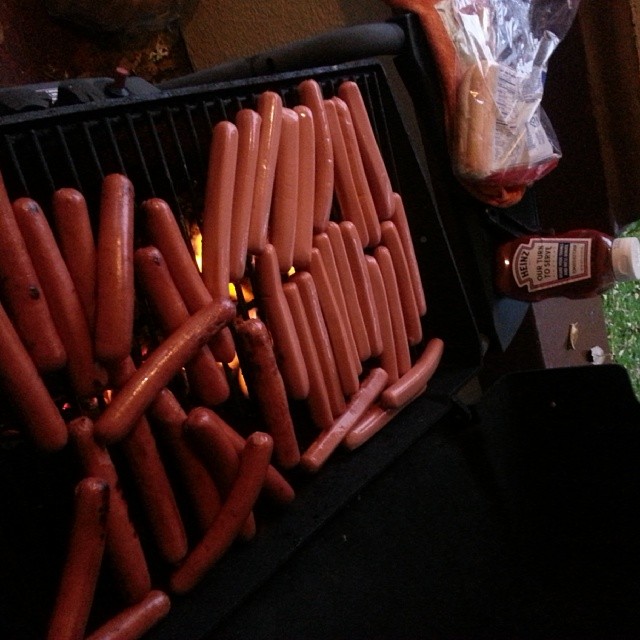This photo depicts an outdoor grill laden with approximately 35 to 40 hot dogs, viewed from a sideways angle, giving the impression the image should be rotated. The black grill is thoroughly covered with hot dogs, some charred and ready to serve, while others appear freshly placed, giving a contrast between cooked and uncooked. The arrangement of the hot dogs varies, some neatly lined up while others crisscross haphazardly. Below the grill, golden-yellow patches of fire are faintly visible. To the side, a Heinz ketchup bottle stands upside down near a plastic bag containing a few white hot dog buns. In the background, a hint of grass is visible, confirming the outdoor setting. Additionally, a small black table is nearby, and the grill features a noticeable red switch at the bottom.